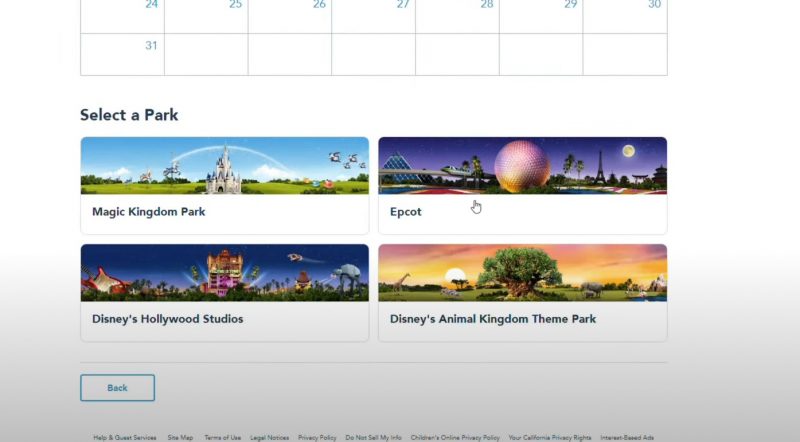The image depicts a section of a calendar with two rows visible at the top. The first row displays dates from 24 to 30 in light blue text, while the second row shows only the number 31 on the left. The calendar grid lines are light gray. Directly below the calendar, in bold black text, is the prompt "Select a Park," followed by four images representing Disney theme parks.

The first image, under the prompt, captures the iconic Cinderella Castle against a backdrop of a blue sky, surrounded by green grass, labeled "Magic Kingdom Park." To its right, the second image features Spaceship Earth, the large geodesic sphere, with a blue sky, a pyramid-like building, a monorail, and palm trees, labeled "Epcot."

Below these, on the left, the third image shows a scene with a guitar, numerous palm trees, and a dark sky, representing "Hollywood Studios." The fourth image, to the right, features a baobab tree and a giraffe against the sky, labeled "Disney's Animal Kingdom Theme Park."